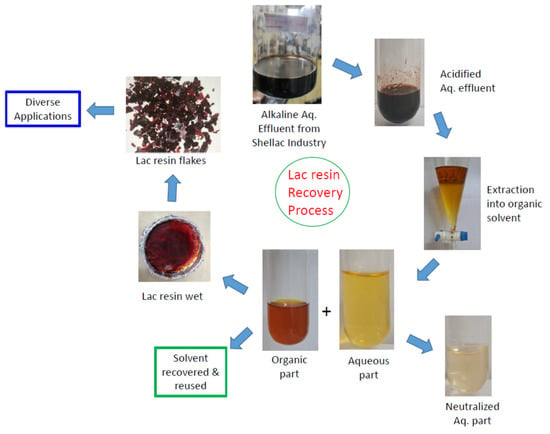This detailed diagram, set on a white background, illustrates the "LAC Resin Recovery Process" prominently in the center, enclosed by a green-outlined circle with white fill. At the top of the diagram is an image labeled "Alkaline AQ Effluent from Shellac Industry," depicting a black liquid in a container. This connects via a blue arrow to the next image on the right, labeled "Acidified AQ Effluent," showing a similar dark liquid. Following this, blue arrows guide the flow to a conical beaker containing a dual-phase liquid labeled "Extraction into Organic Solvent," where the top layer is orange and the bottom is yellow.

From here, the process divides: "Aqueous Part," depicted as a yellow liquid, points to a clear liquid labeled "Neutralized AQ Part." Meanwhile, the orange liquid is labeled "Organic Part," further pointing to a green-outlined square with the text "Solvent Recovered and Reused." This branches to an image of a thick reddish fluid labeled "LAC Resin Wet," which transitions to dark red, nearly black flakes labeled "LAC Resin Flakes." The final step, connected by another blue arrow, leads to a blue-outlined square stating "Diverse Applications."

Complementing these visuals, various connections between the stages are delineated by blue arrows, ensuring a comprehensive understanding of each step in the resin recovery process.